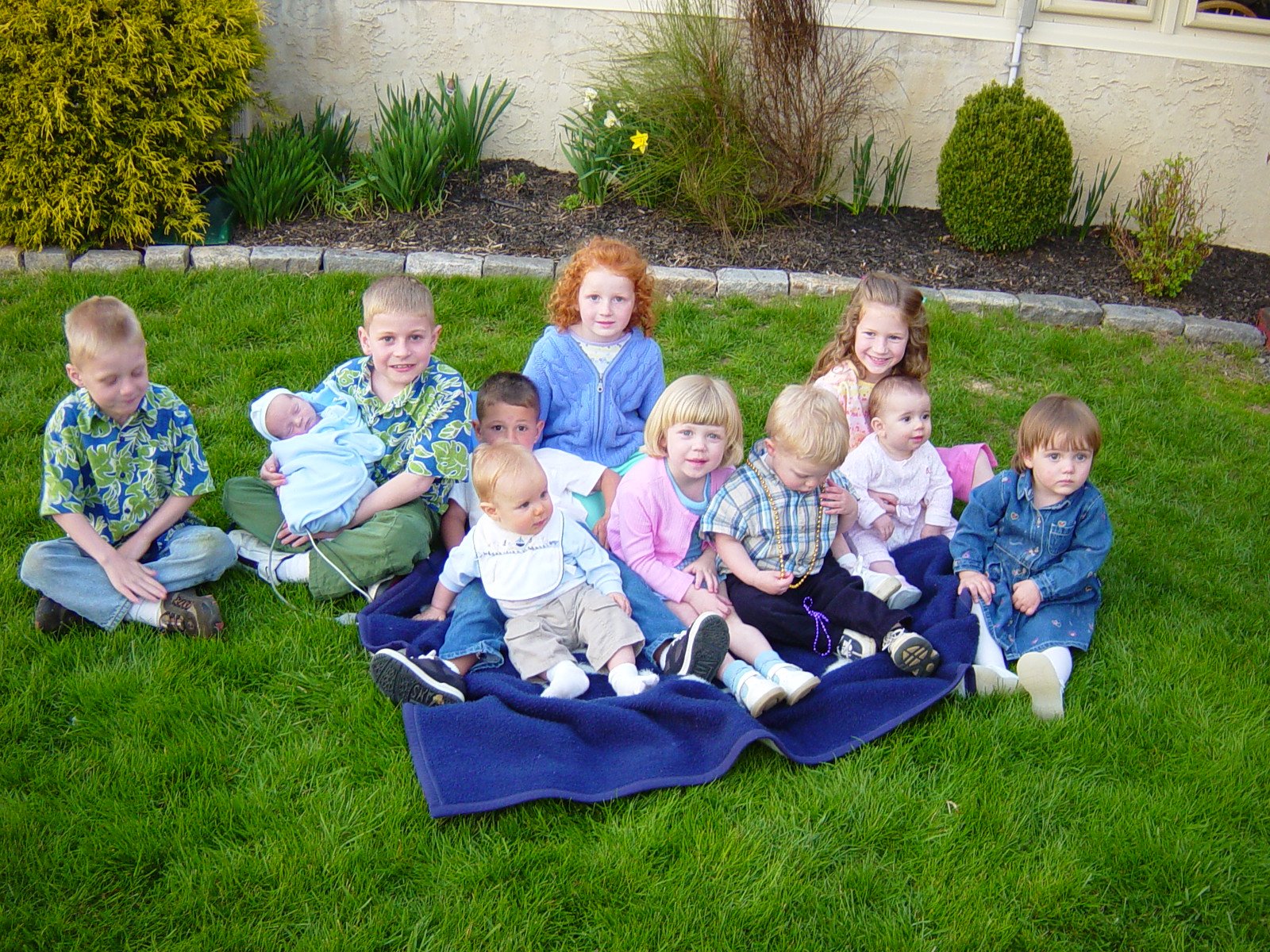In this photograph, a group of around eleven or twelve children, ranging from newborn babies to five-year-olds, are gathered on a verdant lawn, posing for a picture. Most of them are clustered atop a blue blanket that is spread out in the middle of the lush green grass, while a few children prefer to sit directly on the grass. The children display a mixture of reactions; some smile cheerfully while others gaze away from the camera. Attired in a variety of colorful clothing, one child notably wears a blue jersey, and another distinguished by a gold necklace sits centrally. The backdrop features a cream-white textured wall adorned with planted greenery and flowers, including some plants edged with yellow and a central plant boasting a yellow bloom. A small brick pavement runs in front of the wall, adding to the serene garden ambiance of the scene.